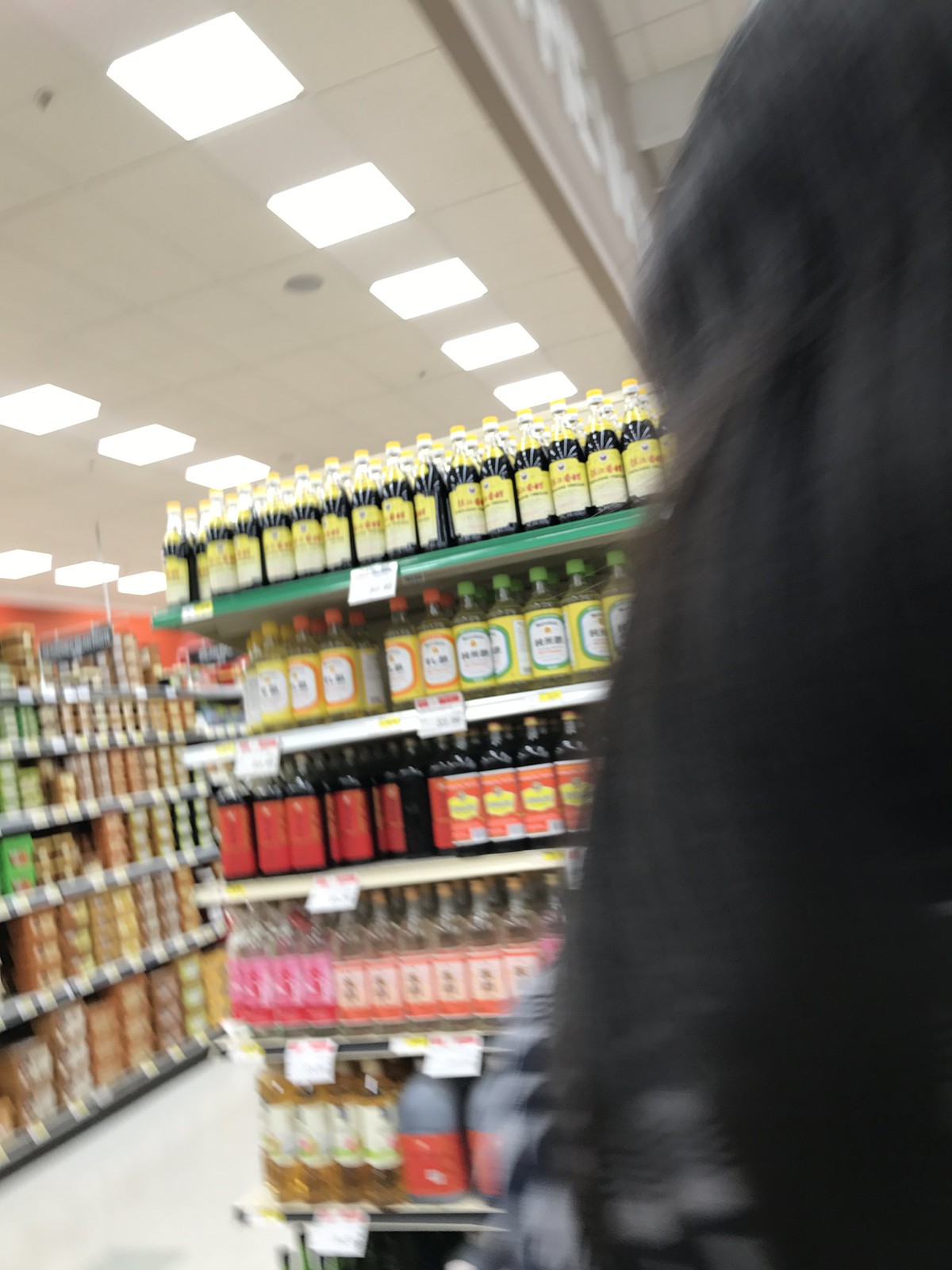The image depicts a well-lit store interior, illuminated by numerous ceiling lights scattered throughout the visible areas, creating a bright and inviting atmosphere. In the foreground, there is a prominently displayed five-tier shelf, fully stocked with merchandise. Each of the five shelves holds multiple jars, all containing various liquids. 

The jars on the top shelf contain a dark-colored liquid, suggesting it might be a type of sauce or similar product. On the second shelf from the top, the jars are filled with a clear liquid. The labels on these jars are predominantly yellow and orange, with white patches that have text displaying the product names.